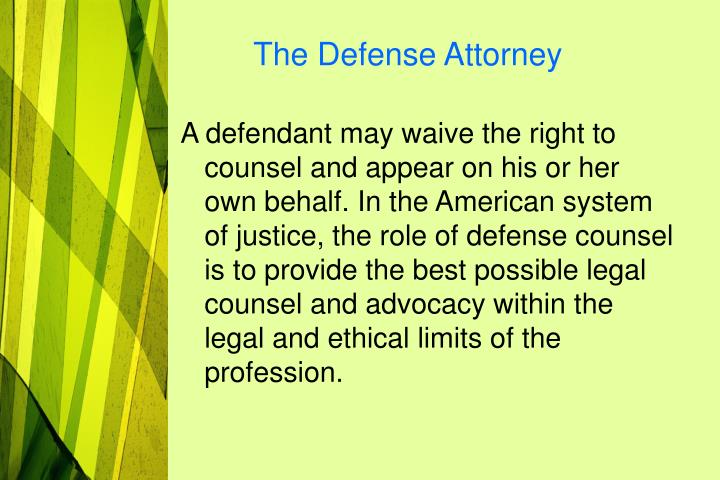The image appears to be an educational slide or study card with a light green background. On the left-hand side, there is a vertically aligned abstract pattern featuring yellow, green, and black plaid stripes, taking up approximately the first third of the image. The top of the slide displays the title "The Defense Attorney" in blue text. Beneath the title is a detailed definition written in black text, stating: "A defendant may waive the right to counsel and appear on his or her own behalf. In the American system of justice, the role of defense counsel is to provide the best possible legal counsel and advocacy within the legal and ethical limits of the profession." The right-hand section, which comprises about three-quarters of the background, is filled with a lime green hue. This suggests the slide is likely intended for educational purposes, possibly as study material for students.